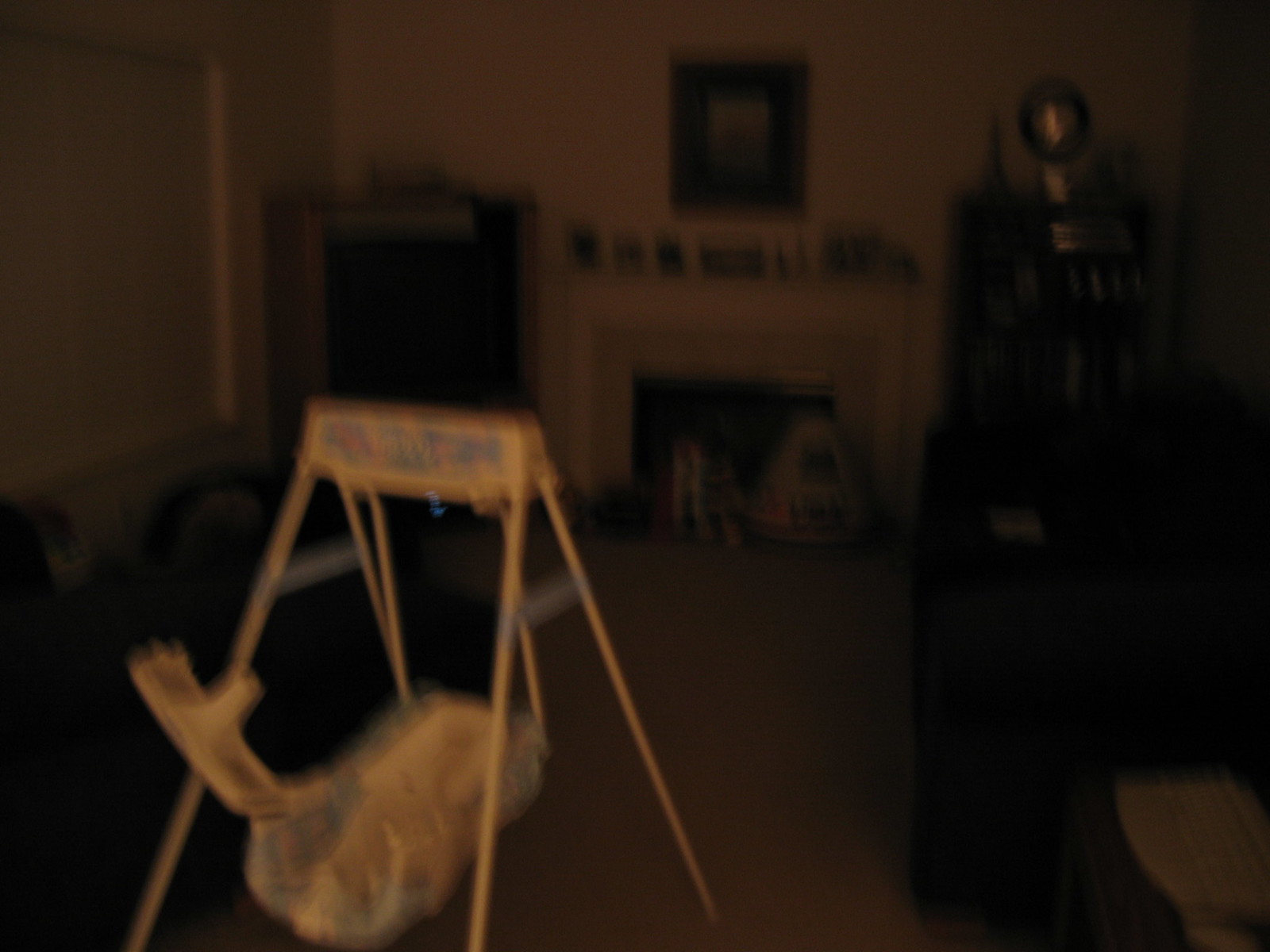The photograph depicts a dimly lit indoor front room of a home, primarily centered around an unlit black rectangular fireplace. Above the white mantle of the fireplace, a painting or picture is discernibly hung, contributing to the room's decor. The mantle itself holds several indistinct items due to the blurry and grainy nature of the photo, which is exacerbated by low light conditions.

On either side of the fireplace, there seem to be pieces of furniture — likely dark brown cabinets or bookcases, one of which might host a large ball-shaped trophy and an additional clock. The walls of the room are white, contrasting with what appears to be light gray carpet covering the floor, though the poor lighting makes color distinction difficult.

Prominently in the foreground, positioned to the left, is a white baby swing featuring a cradle area intended to soothe or rock a baby to sleep. The swing has accents of blue, with a rectangular piece at its top that includes some pink and blue colors and writing, though the specifics are not clear. The swing's support structure consists of two bipod pairs of legs. The overall image is slightly blurred, making finer details fuzzy but still offering a glimpse into this cozy living space.